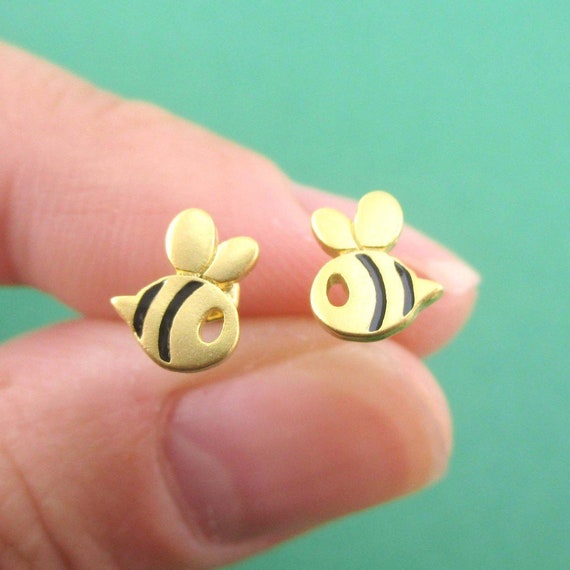The image showcases a light teal background with a close-up of someone's thumb and forefinger holding a pair of stud-style earrings. The fingernails are plainly visible, bearing no polish, while the earrings are the focal point, rendered in sharp detail. The earrings are small, designed in the shape of bumblebees. They feature a gold base color with two black stripes on their bodies and a teardrop shape. Notably, each bee's eye is depicted as a hollow circle. The bees appear to be facing each other, adding to their charming and cute aesthetic.